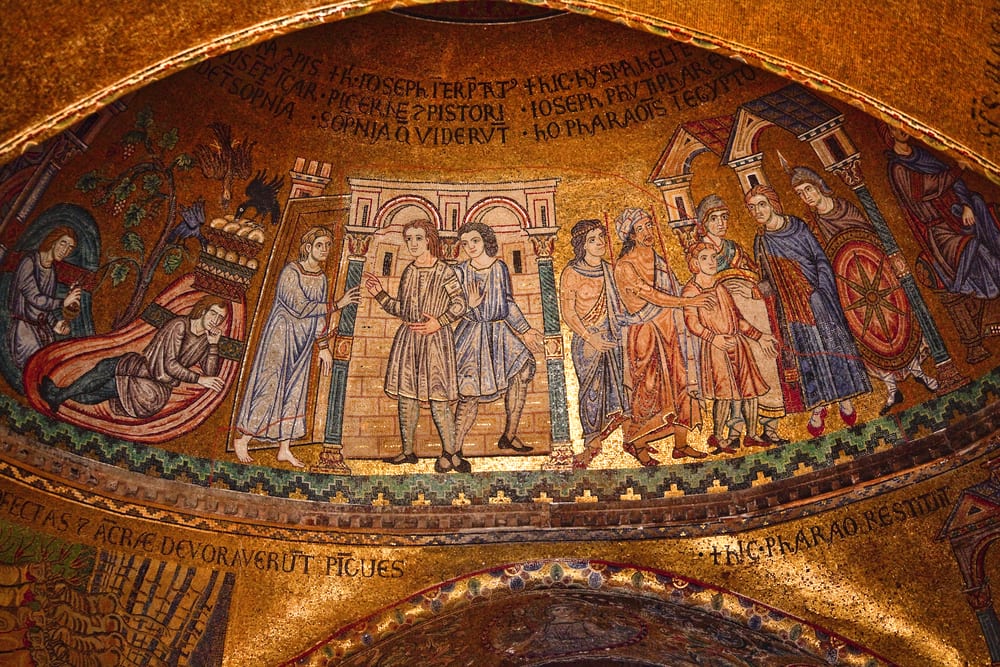The image captures a highly detailed, realistic photograph of the interior ceiling of a basilica, showcasing an ornate, gold-colored mural. The scene within the mural is rich with historical and religious iconography, likely inspired by Roman or Byzantine art. The mural is divided into several intricate scenes featuring multiple figures adorned in blue, gray, and red robes, reminiscent of medieval or ancient attire. At the center, a couple of people stand out, with a depiction of a cityscape and brick walls in the background. Black text, possibly in Greek or Latin, is inscribed above and below the mural. The narrative unfolds with three soldiers on the right, receiving a young boy from three other figures, while the center captures two individuals waving, with one pointing towards another. On the far left, two people are seen lounging, one with what appears to be food on their head, attracting several black birds, adding to the rich tapestry of this visually stunning piece. The surrounding structure complements the mural with arches along both the top and bottom, enhancing the grandeur of this religious or governmental edifice.